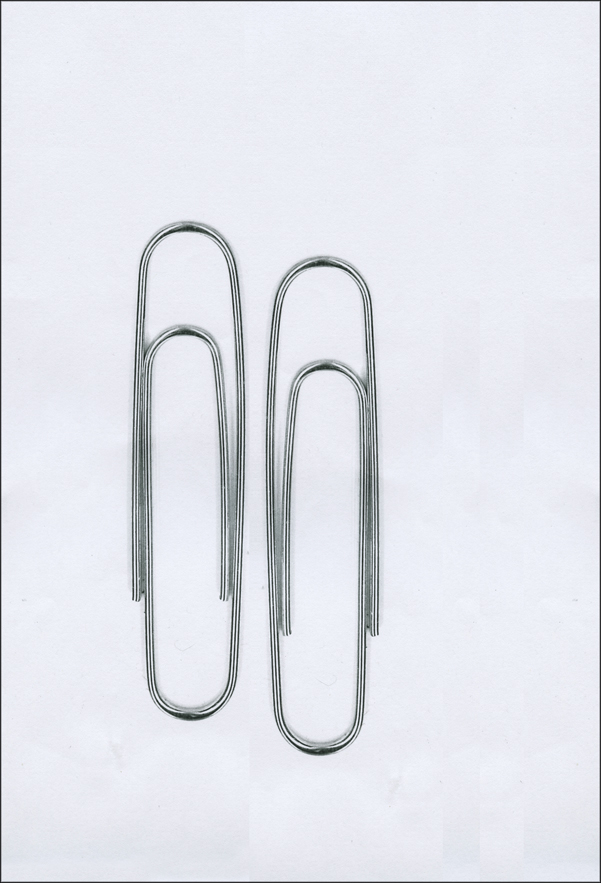The image depicts a stark, minimalist composition featuring two oversized, silver-gray paperclips set against a white backdrop. The highly zoomed-in photograph gives the impression that the paperclips are monumental, approximately five feet tall if they were life-size. These standard, rounded paperclips are positioned side by side with one slightly higher than the other, enhancing the simple yet striking visual arrangement. The simplicity of the scene underscores its artistic appeal, leaving it ambiguous whether it is a piece of art or a meticulously composed photograph.